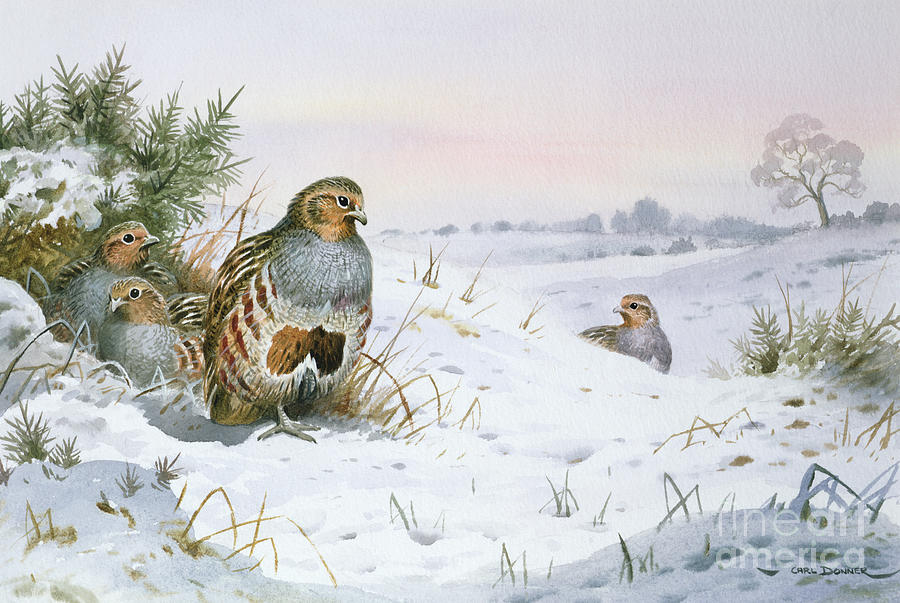The painting depicts a serene snowy field bustling with a small family of pheasants. At the center, a mother pheasant, characterized by her brown and white feathers, stands watchfully over her three younglings. Two of the chicks nestle closely behind her, basking in the warmth and security of their mother's presence. The third chick, however, curiously pokes its head over a small hill nearby, yet remains within a safe distance. The ground is blanketed in pristine white snow, with patches of grass in varying shades of green and yellow breaking through the frost, suggesting a mixed terrain of thriving and withered flora. 

Directly behind the mother and the two chicks, there appears to be clumps of grass, hinting at a potential nesting area. In the distance to the right side, a tree stands tall, accompanied by a faint row of other trees subtly blending into the horizon. The sky is light with a pinkish tint, suggesting an early morning or late afternoon glow, casting a soothing ambiance over the scene. The painting captures a moment of natural unity and watchfulness, with the mother pheasant's watchful eyes ensuring the safety of her adventurous youngling while maintaining the tranquility of the wintry landscape.